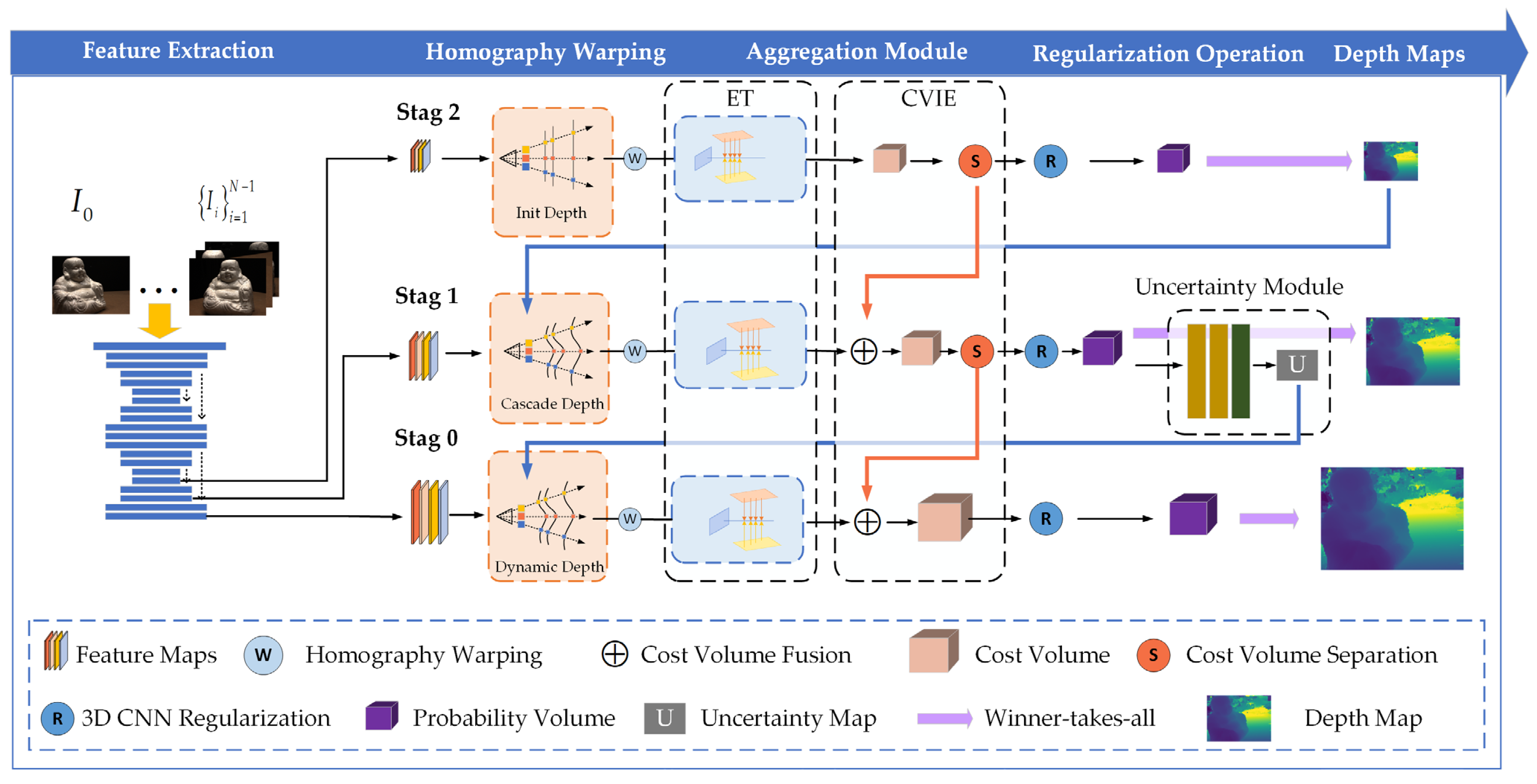The image is a detailed diagram with various symbols, arrows, and labels situated against a white background. At the top left, it begins with the text "feature extraction" in white letters. Moving rightward, the labels "homography warping," "aggregation module," "regularization operation," and "depth maps" follow sequentially. Below these headings, the diagram is divided into sections, each containing different graphical elements, such as a beige square with arrows, a blue square featuring a yellow and beige device, and various interconnected shapes and symbols.

For example, near the center, there are two photos of a Buddhist statue linked by a yellow arrow pointing downwards. This leads to a series of blue lines with cascading arrows that further connect to different symbols, such as colored papers arranged by size. One of the notable elements is the bottom row label "stag zero," which branches out to terms like "dynamic death" and follows a complex path through various stages marked by shapes including a W, a series of lights, a "+" sign, a cardboard box labeled "cost volume," an R, a purple cube, and an inverted colored photograph labeled "depth map."

Lower in the diagram, there are additional labels like "feature maps," "homography warping," "cost volume fusion," "cost volume," "cost volume separation," "3D CNN regularization," "probability volume," "uncertainty map," and "winner takes all." Red arrows connect elements labeled with the letters S and R, with S in red and R in blue. The bottom section of the diagram provides a legend explaining the different shapes and their meanings, ensuring the viewer can decode the complex relationships and processes depicted in the image.